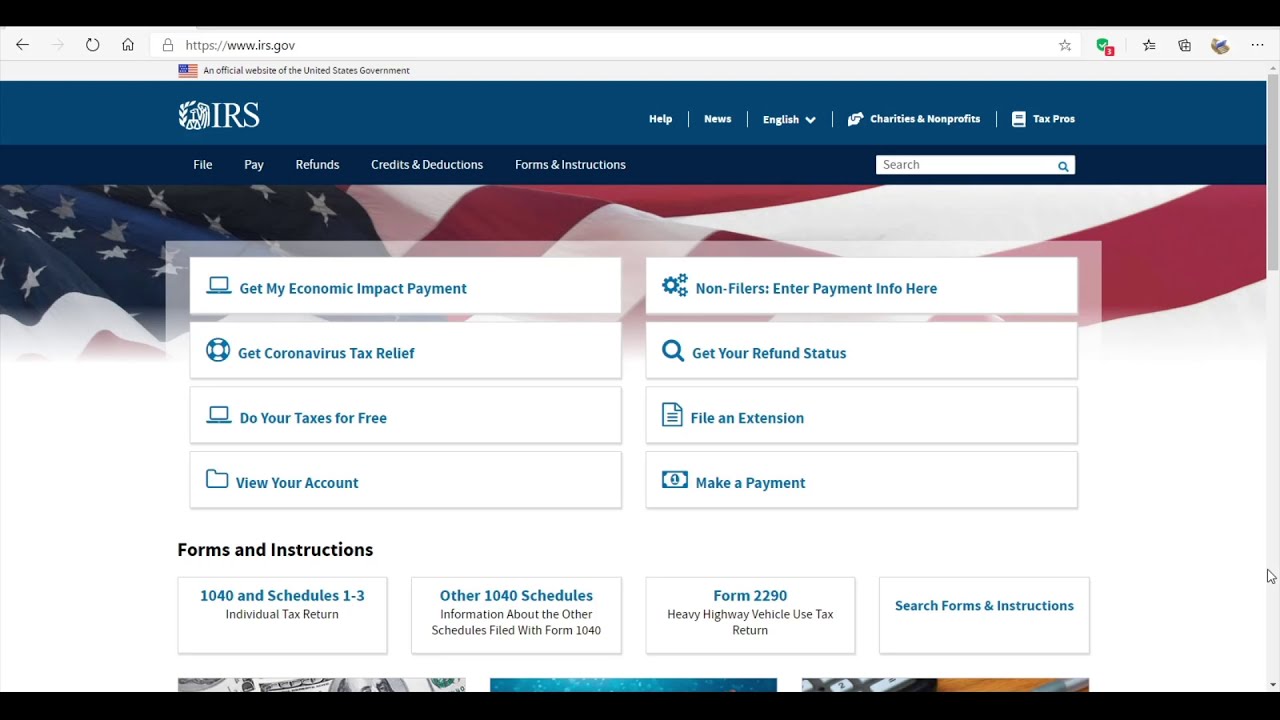Screenshot of the IRS Website Homepage:

The screenshot captures the visible portion of the www.irs.gov website on a desktop or laptop computer. At the very top, the browser interface is visible with typical navigation options, including back, reload, and home buttons, indicating that the site is being accessed in secure mode.

The webpage features a distinctly structured layout:
1. **Header Section**:
   - The topmost section displays a blue bar with the IRS logo and key links for navigation.
   - Below the blue bar is a darker blue secondary bar which hosts additional navigational tabs or actions.
   - An American flag icon is prominently displayed, gently waving.

2. **Navigation Menus**:
   - The first blue bar provides primary options such as Health, News, Language selection (defaulted to English), Charities & Nonprofits, and Tax Pros.
   - Beneath this, a secondary menu bar allows users to easily access sections like File, Pay, Refunds, Credits & Deductions, and Forms & Instructions. This bar also includes a search bar for quick site-wide searches.

3. **Main Content Area**:
   - The content area features a clean white background, populated with multiple entries or links catering to specific actions. These include Economic Impact Payment, Refund Status, Coronavirus Relief, Free Tax Filing options, Filing Extensions, Account Viewing, and Payment Making.
   - Additionally, forms and instructions are accessible to guide users through various processes. The page structure suggests that more content is available upon scrolling down.

The overall design incorporates a mix of blue gradients and a straightforward layout, ensuring easy navigation and accessibility for all users seeking IRS-related information and services.